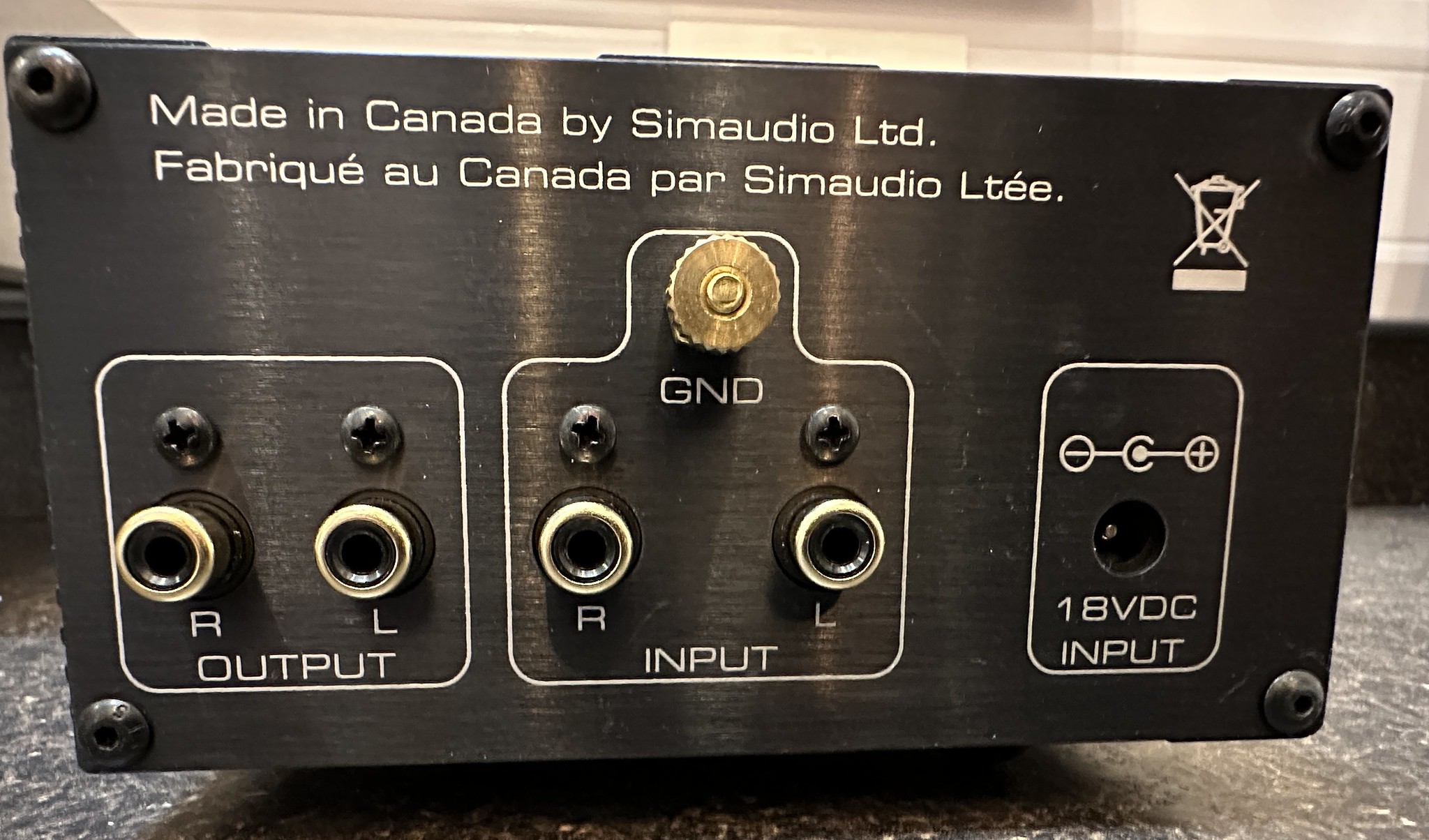This photograph captures a close-up view of the back panel of a dark gray, rectangular, metal amplifier, which is poised on a black floor with beige splatterings. The equipment is a robust unit manufactured by Simaudio Ltd., as indicated by the text “Made in Canada by Simaudio L-T-D” etched at the top, paralleled by its French translation, “Fabrique Canada par Simaudio L-T-E-E.” The surface of the amplifier features four rivets securing the back panel, with additional bolts on each corner.

Central to the design is a gold-colored button labeled “GND.” The panel also exhibits a series of rounded square ports marked for inputs and outputs, specifically designated with "R" for right and "L" for left. Accompanying these ports is an 18-volt DC input, with clear positive and negative indicators. The overall impression is one of meticulous craftsmanship, underscoring both functionality and aesthetic finesse in audio equipment design.